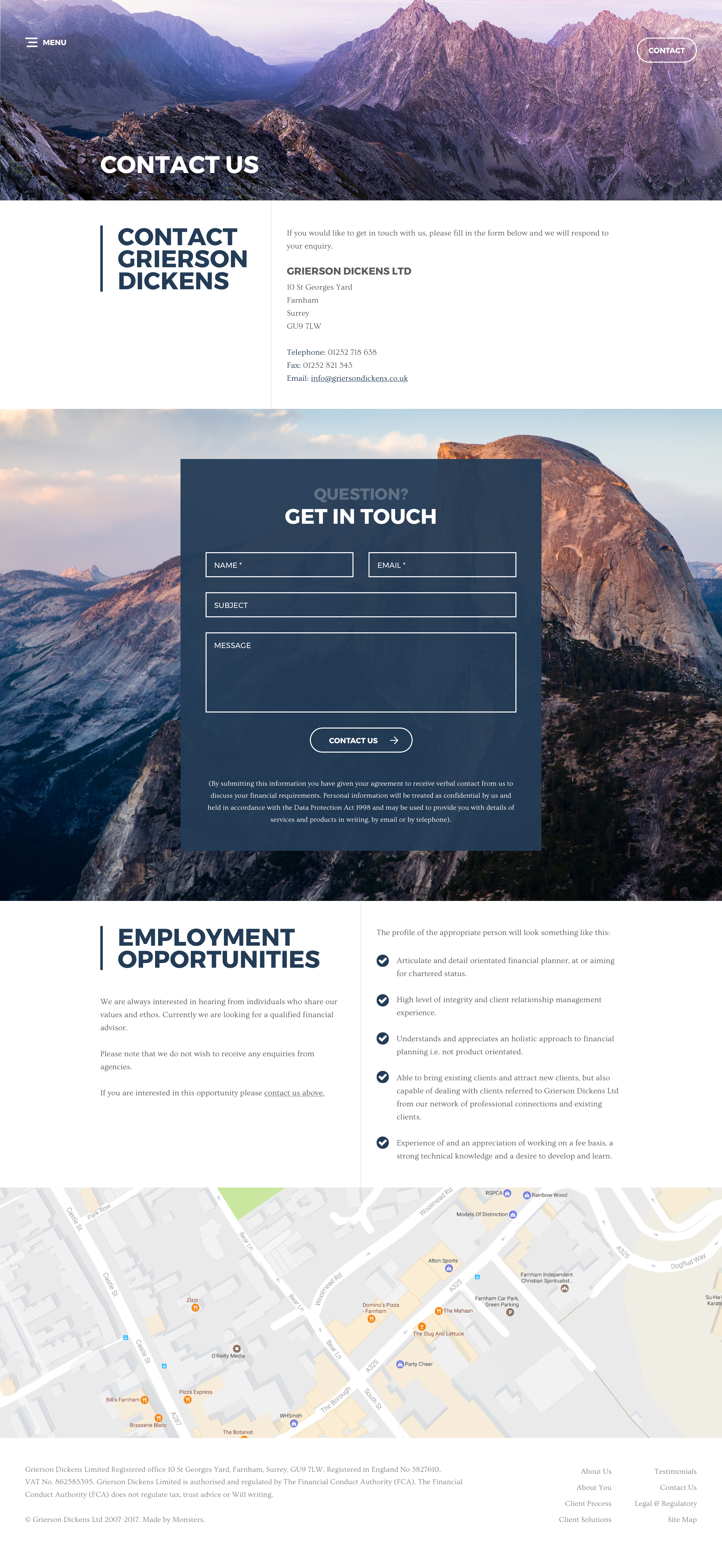The image depicts a visually appealing website featuring a stunning mountain landscape with varying lighting – some peaks basking in sunlight while others lie in shadows. A serene valley runs between these majestic mountains. Dominating the scene, large text sprawled across one of the mountain faces reads "Contact Us." Just below, in smaller print, it states "Contact Grierson Dickens," followed by a portion of exceedingly small text, difficult to discern.

Beneath this is a distinct, closer image of another mountain range. This secondary image is overlaid with a dark gray box prominently inscribed with the words "Get in Touch" in an easily readable font. Above this prominent message, the word "Question" appears in a washed-out gray color. The gray box includes fields for users to input their name, contact details, and message or query in a larger text area.

Further down the page, the text "Employment Opportunities" appears along with a series of bullet points, though this text is also too small to be legible. At the very bottom of the page, a faintly colored map is included, marked with labels and towns that are unfortunately too minuscule to be read clearly.